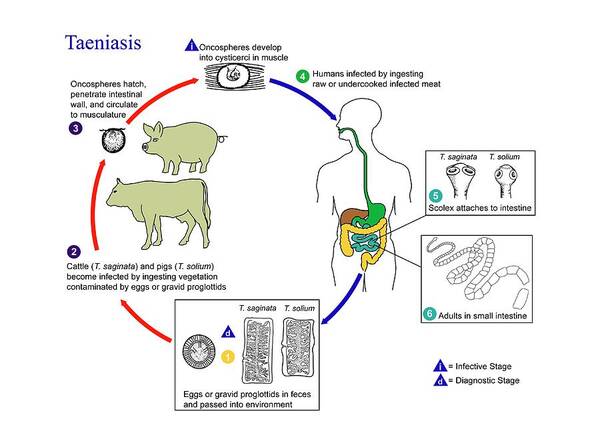This image is a detailed, horizontally aligned scientific diagram, likely from a biology textbook, depicting the life cycle of the parasite Taenia (teniasis). The title "TAENIASIS" is prominently displayed in large, blue Times New Roman font at the top left. The diagram features a roughly oval shape with arrows traversing a clockwise pattern, illustrating the parasite's developmental stages.

At the upper left, there is an illustration of a pig and a cow, annotating their role in the life cycle. Directly below this, a text box indicates the initial stage: "Oncospheres hatch, penetrate the intestinal wall, and circulate to musculature." Adjacent to this is a close-up of a spiral-shaped form, likely representing the early development of the parasite.

The diagram continues to the right where a blue triangle (with a white "I") denotes the infective stage, showing the parasite's development in muscle tissue. Next, a green circle (marked "4") highlights the stage where humans become infected by ingesting raw or undercooked infected meat, with a detailed outline of the human digestive system and anatomical symbols identifying the various internal organs, including the stomach and intestines.

Adjacent to the human figure, there are finely rendered images of the parasite's head and respective body components (labeled "T. saginata" and "T. solium"), indicating different species. This segment is also marked with a teal circle labeled "5," signifying the stage where the scolex (head) attaches to the intestines.

Moving down, the diagram notes "Adults in the small intestine" next to another finely detailed representation of the parasite. There is a teal circle (marked "6") indicating the final development stage within the human host. Another text box reads, "Eggs or gravid proglottids in feces and passed into the environment," highlighting the completion of the life cycle.

To the left, a segment where arrows guide viewers to visualize cattle and pigs becoming infected by consuming vegetation contaminated with eggs or gravid proglottids is marked by a navy blue circle labeled "2." The description for the infected animals is annotated specifically for cattle (T. saginata) and pigs (T. solium).

Throughout the diagram, a legend at the lower right aids in interpreting symbols with blue and red arrows indicating different stages of the cycle, including infective and diagnostic stages, denoted by small triangles and text.

Overall, the image intricately details the life cycle of the parasite Taenia, emphasizing each stage of development through clear, sequential illustrations and comprehensive annotations.